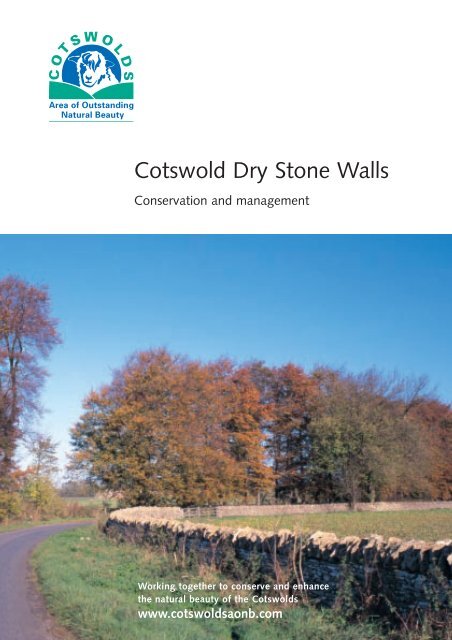This advertisement showcases the natural beauty of the Cotswolds in a fall scene. Dominated by a predominantly clear, blue sky, the central image features a scenic meadow dotted with trees that exhibit brilliant hues of orange, red, yellow, and brown, indicative of the autumn season. A well-maintained, gently curving dry stone wall made of various shades of gray stone stretches across the landscape, starting from the bottom right corner and looping back to the right, enveloping a vibrant green grass field on either side. A dark gray paved road appears on the left, offering a serene contrast to the natural elements, and a solitary red-leafed tree stands distinctly on the far left. 

At the top of the advertisement, set against a white background, is a logo featuring a blue line drawing of a shaggy lamb with a glowing blue sun in the background. Above this logo, the word "Cotswolds" arcs in green text, with two green hills positioned below the lamb. Below the image, black text reads, "Cotswold Drystone Walls, Conservation and Management," underlining the theme of preservation. Centered at the bottom, white text emphasizes the core message: "Working Together to Conserve and Enhance the Natural Beauty of the Cotswolds." The website URL, www.cotswoldsaonb.com, is provided for further information.